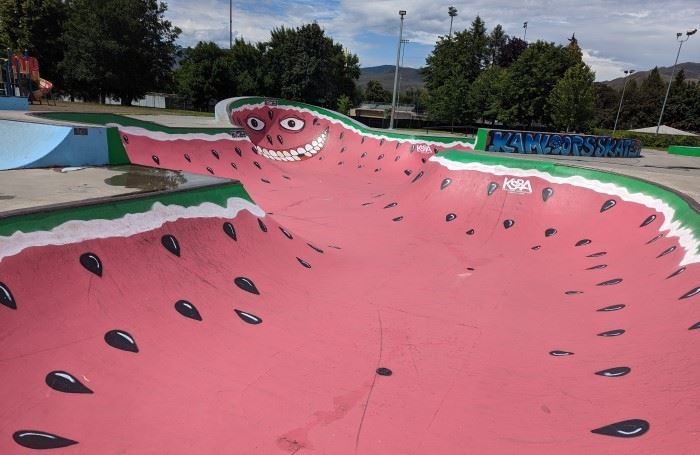The image depicts an outdoor skating park bathed in daylight, framed by a sky of light blue and dotted with puffy white clouds. In the background, green trees and light poles line the scene, marking the boundary of the park. The sky cascades down to a picturesque mountain range. Scattered light poles provide a hint of the park’s infrastructure, suggesting it's a well-maintained recreational area. The central focus is a large ramp intricately painted to resemble a watermelon; the outer edge is green with a white stripe, transitioning into a red interior complete with black seeds. This vibrant ramp also features a smiling face near its top. On the right side of the image, a partially visible blue ramp accentuates the playful nature of the scene. A sign with blue letters reads "skate," although it's not prominently positioned. The colors within the scene range from varying hues of green and blue to pops of red, black, and white, enhancing the lively and inviting atmosphere of the skating park.